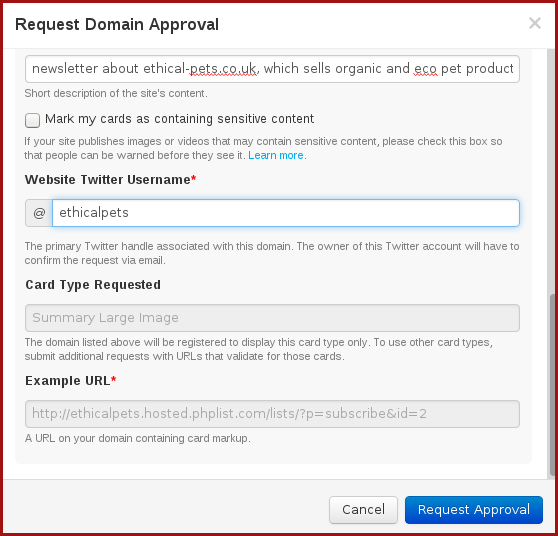This image is a vertical screenshot of a web page designed for submitting a request for domain approval. The page is bordered by a reddish-maroon box, providing a distinct frame to the content within. 

At the top of the page, there is a white background with the heading "Request Domain Approval" in bold black text. Following this, there is a gray box overlaid on the white background. Within this box is a search bar containing the text "newsletter about ethicalpets.co.uk," indicating that the site sells organic and eco-friendly pet products. Beneath the search bar, a short description invites users to provide details about the site's content.

Below the description, there is an unchecked checkbox next to the text "Mark my cards as containing sensitive content." Accompanying this is a brief message advising users to check the box if their site publishes images or videos that may contain sensitive content so viewers can be warned appropriately. Adjacent to this message is a blue "Learn More" button.

Further down, a section titled "Website Twitter Username" in bold black text follows. A red asterisk indicates that this field is mandatory. The provided example is "@ethicalpets" within a search bar, signifying the primary Twitter handle linked to the domain. A note explains that the owner of this Twitter account will need to confirm the request via email.

Next, the section "Card Type Requested" is emphasized in bold black text. It specifies "Summary with Large Image" as the requested card type, suggesting that the domain listed will only be registered to display this specific card type. Users are instructed to submit additional requests for other card types, ensuring each request URL validates accordingly.

There is also an "Example URL" field marked with an asterisk, featuring the text "URL on your domain containing card markup." At the bottom of the page are buttons for "Cancel" and "Request Approval," allowing the user to either abort or proceed with their domain approval request.

Overall, the text and layout are clear and user-friendly, guiding the user through the necessary steps to request domain approval effectively.